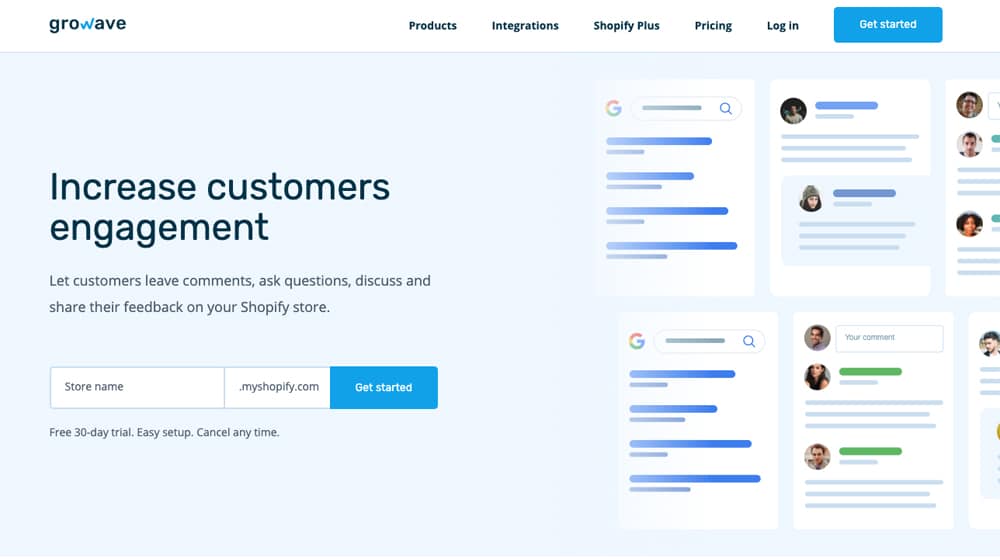This is an image of the Grow Wave website homepage. In the top left corner, the Grow Wave logo is prominently displayed. The "GRO" portion of "Grow" is in blue and the "W" is also in blue, while "WAVE" is rendered in black, in a different font style. The logo is situated within a white top menu bar that spans horizontally across the page. 

The top menu includes several navigation links: "Products," "Integrations," "Shopify Plus," "Pricing," and "Login." At the far right of the menu, there's a blue "Get Started" button with white font.

Below this menu bar, on the left side, the heading "Increase Customer Engagement" is written in large black font. Underneath this headline, a smaller black font provides additional details: "Let customers leave comments, ask questions, discuss, and share their feedback on your Shopify store."

Beneath this text, there are two input boxes. The first box is labeled "Store Name," followed by ".myshopify.com." Next to these boxes, a blue "Get Started" button with white font offers a call-to-action for visitors.